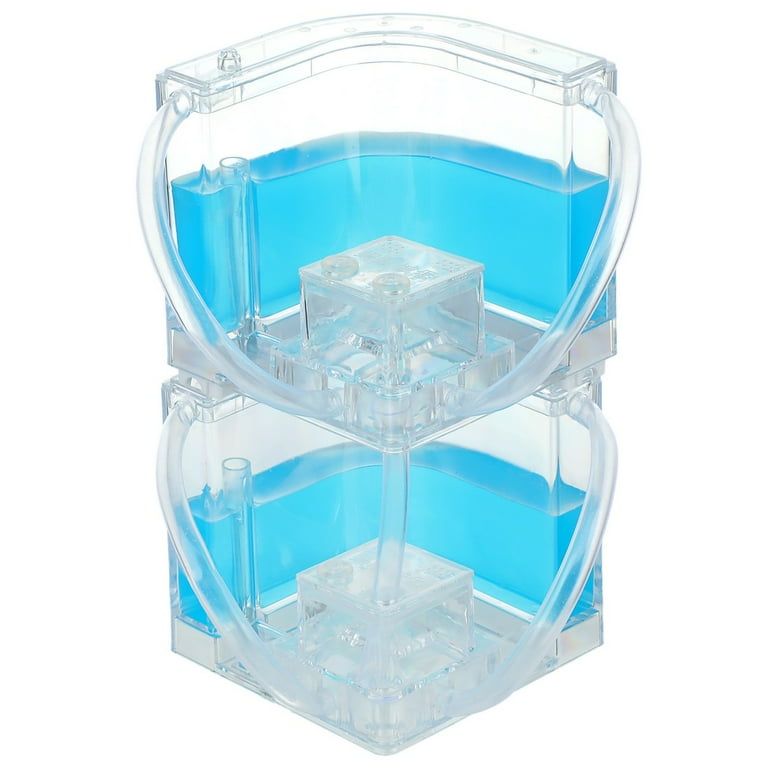The image showcases a geometric, cube-shaped structure made of a clear, glass-like plastic, filled with a bright, turquoise fluid that appears very cleansing and refreshing. The structure is composed of several interconnected sections: a central, silver or gray cube, and two larger transparent squares stacked vertically with tubes connecting each part, allowing the fluid to flow between them. The structure stands against a white background, emphasizing its sleek, modern design, typical of product imagery. The overall palette includes shades of aqua blue, white, and gray.